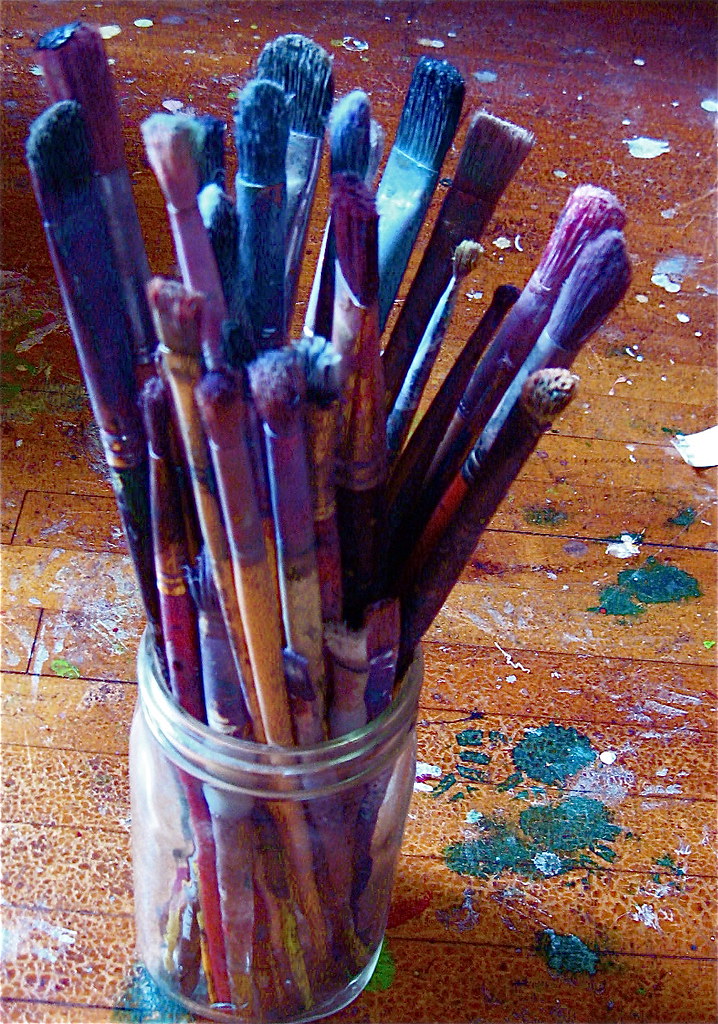The photograph captures a clear jar filled with a dozen paintbrushes, resting on a brown, wooden floor heavily splattered with a variety of paint colors, including white, green, dark aqua, and blue. The jar, which has distinct grooves around its top, holds paintbrushes of varying sizes and shapes—some with straight bristles and others with rounded bristles. Each paintbrush is coated in shades of dark blue and purple paint, suggesting they have either just been used or have not been cleaned in a while. The paintbrush handles are diverse in color, featuring hues of yellow, reddish-pink, and natural wood. The wooden floor beneath them is marked with numerous paint splotches, indicating a busy and colorful painting environment.